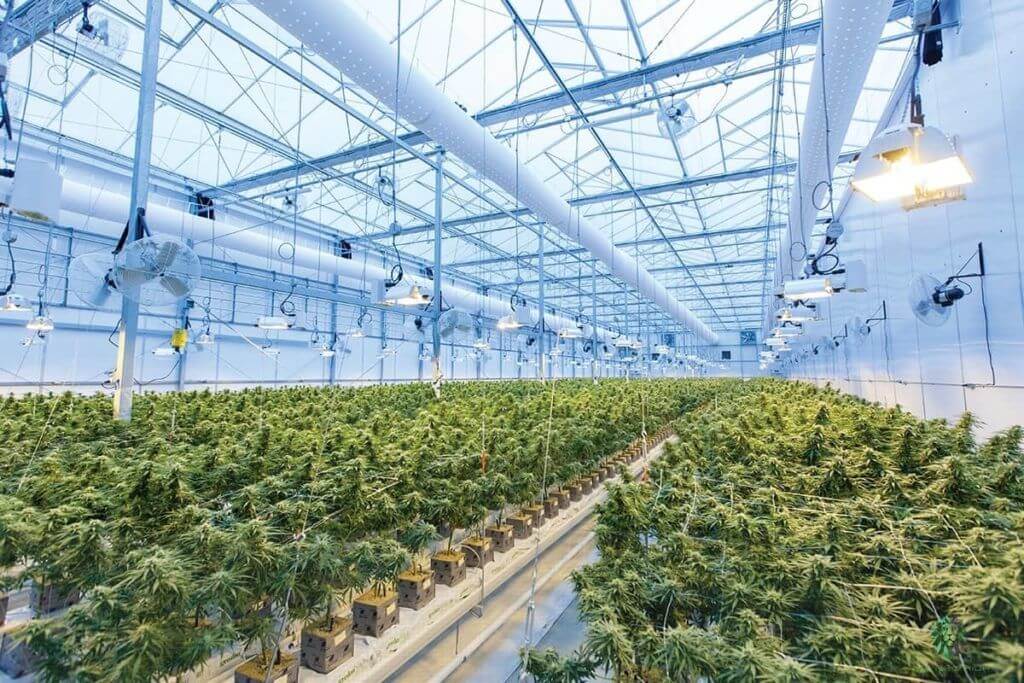The image depicts an expansive industrial-sized greenhouse with rows upon rows of marijuana plants densely packed along the floor. The greenhouse interior features a network of large, square-netted structures suspended over the plants, providing support and perhaps aiding in their growth. Amidst the greenery, a central walkway runs through the greenhouse, offering a path to navigate between the lush rows.

The ceiling, painted white and constructed with metal frames, is lined with a combination of hanging lights and heat lamps, casting a striking bluish and yellowish glow onto the pristine vegetation below. Ventilation pipes and ceiling-mounted fans are strategically placed down the length of the greenhouse, ensuring optimal air circulation. Additionally, fans are mounted on poles along the side walls, evenly spaced to maintain a consistent climate throughout the space.

The plants themselves burst with various shades of green, illuminated under the specialized lighting, revealing a vibrant tableau of dark and light greens. This meticulously designed environment optimizes the growth conditions for the thousands of marijuana plants cultivated within this extensive indoor growing area.